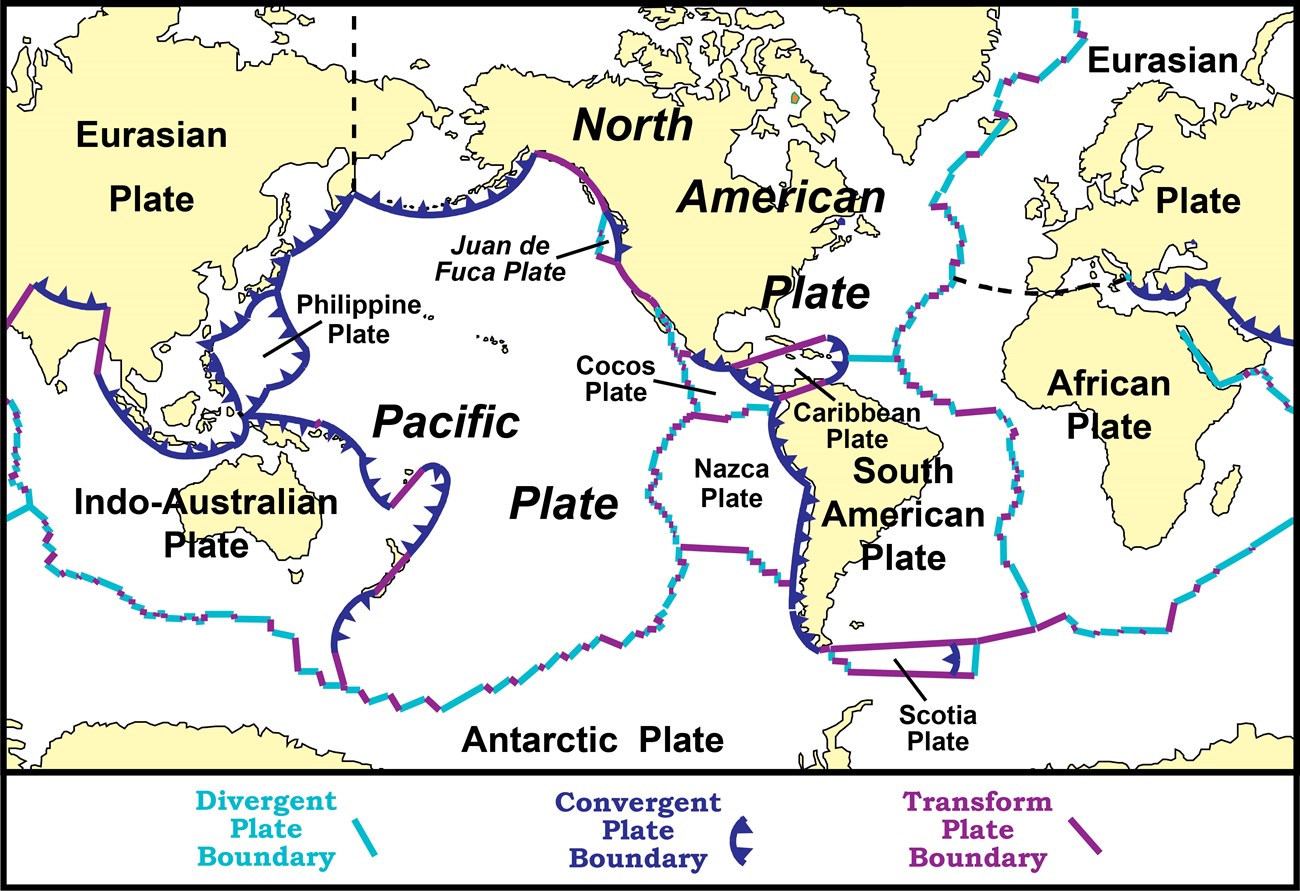This image is a detailed, colorful map of Earth's tectonic plates, laid out in a square format. The map features all the major tectonic plates, including the Eurasian plate, North American plate, African plate, South American plate, Antarctic plate, Pacific plate, Australian-Indian plate, Philippine plate, Cocos plate, Caribbean plate, Juan de Fuca plate, Scotia plate, and Nazca plate. The continents are shaded in light yellow, while the oceans are white, highlighting the intricate boundaries of the tectonic plates.

Different colored lines represent various types of plate boundaries: light blue lines indicate divergent plate boundaries, darker blue lines show convergent plate boundaries, and purple lines mark transform plate boundaries. Some boundaries feature multiple colors to represent areas where more than one type of boundary interaction occurs.

A legend at the bottom of the map clarifies the meaning of these boundary lines: light blue for divergent boundaries, dark blue for convergent boundaries, and purple for transform boundaries. This map provides a comprehensive overview, with the continental plates depicted transcending land borders into the ocean, illustrating the dynamic nature of Earth's lithosphere.